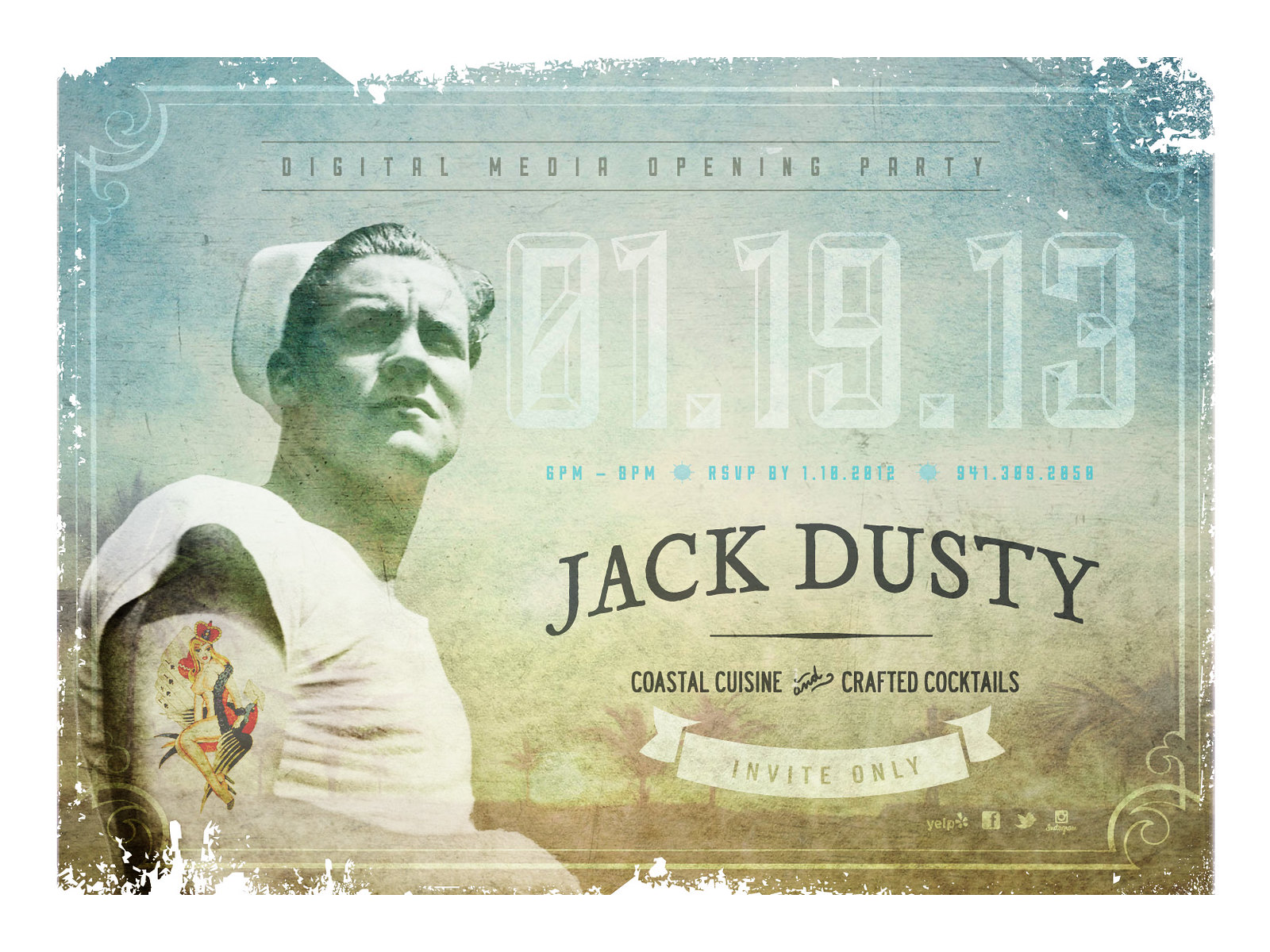This advertisement, evocative of a vintage poster, features a scuffed and faded cardboard background with chipped coloring around the edges. The image is divided into a gradient of pale blue at the top to light brown at the bottom. On the left side of the square is a tinted black-and-white photo of a sailor—an older white man gazing into the distance, wearing a white t-shirt and sailor hat, with a colorized tattoo of a blonde mermaid on his upper arm. 

Across the top of the advertisement, in small letters, it reads "Digital Media Opening Party 01-19-13" with the event time of "6pm to 8pm" in blue lettering below that. The main focus is the large black uppercase text, "Jack Dusty," with "Coastal Cuisine with crafted cocktails" in a smaller font beneath it. The final detail, "Invite Only," is prominently displayed across a ribbon at the bottom of the image, highlighting the exclusivity of the event. The overall aesthetic, with its blend of vintage elements and intriguing visuals, suggests a nostalgic yet sophisticated atmosphere for an exclusive gathering.